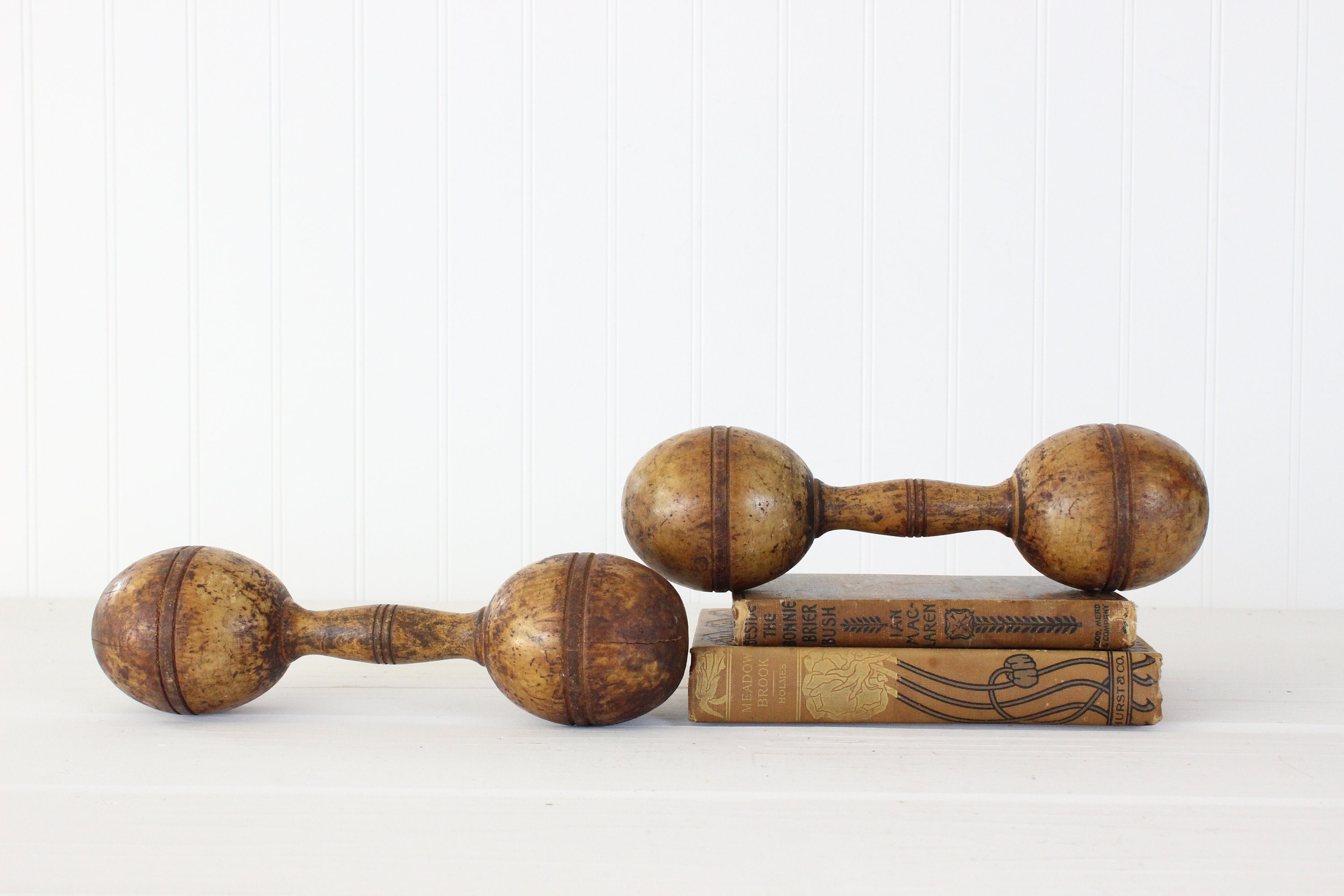In the image, there are two wooden maracas, which resemble barbells with hollow, bulbous spheres on each end connected by a stick. These maracas, filled with beads, are designed to produce a rattling noise when shaken. The scene is set against a white background with a white table. 

On the right side of the image, there are two tan books laying flat and stacked on top of each other. The bottom book has "Meadowbrook" written on its spine with a floral design, while the spine of the top book reads "Beside the Awni Brer Bush." One of the maracas rests on top of these books. The second maraca is positioned to the left of the books, directly on the table. There are slight shadows cast by the maracas and the books, adding depth to the composition.